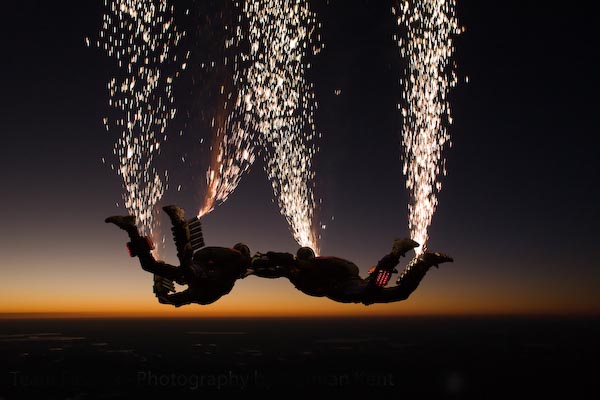The image captures a pair of skydivers free-falling through the evening sky, with the descending sun casting a warm glow and hinting at dusk. The skydivers, suited up in full gear including helmets and parachutes, are holding onto each other as they plummet high above the earth. Attached to their ankles are devices emitting vibrant sparks and flames, resembling a fireworks display. These pyrotechnic tubes create a dazzling spectacle against the backdrop of the darkening sky. The photograph, although marked with a partially obscured watermark reading "photography," vividly portrays this dramatic descent with sparkling trails illuminating the scene, emphasizing the adventurous and visually stunning nature of the moment.